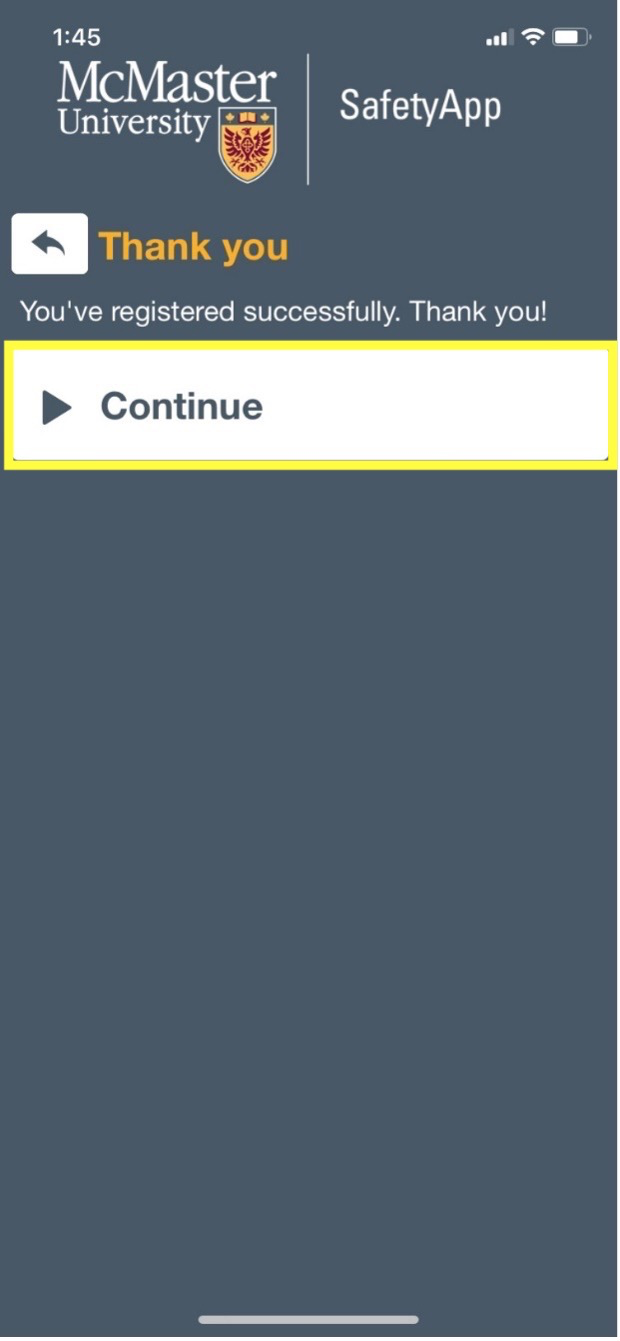This image is a detailed screenshot from a cell phone set against a dark gray background. In the upper left corner, the time reads "1:45," and the upper right corner shows three out of four bars of reception along with a lit Wi-Fi icon. The battery indicator displays nearly full charge.

Prominently positioned below is a gold shield icon with a white border and black accents on the top. Inside the shield, there is an illustration of a red eagle-like bird. Above the eagle's head, a gold-colored book is flanked by two maple leaves, one on each side.

In the upper left corner of the screenshot, "McMaster University Safety App" is displayed in clear, bold text. Below this, large gold print says "Thank You" with an accompanying arrow in a box, indicating successful registration. Underneath it, white text confirms, saying, "You've registered successfully, thank you."

At the bottom of the screenshot is a box bordered in bright yellow. Inside this white box is black text that reads, "Continue," accompanied by an arrow pointing to the right.